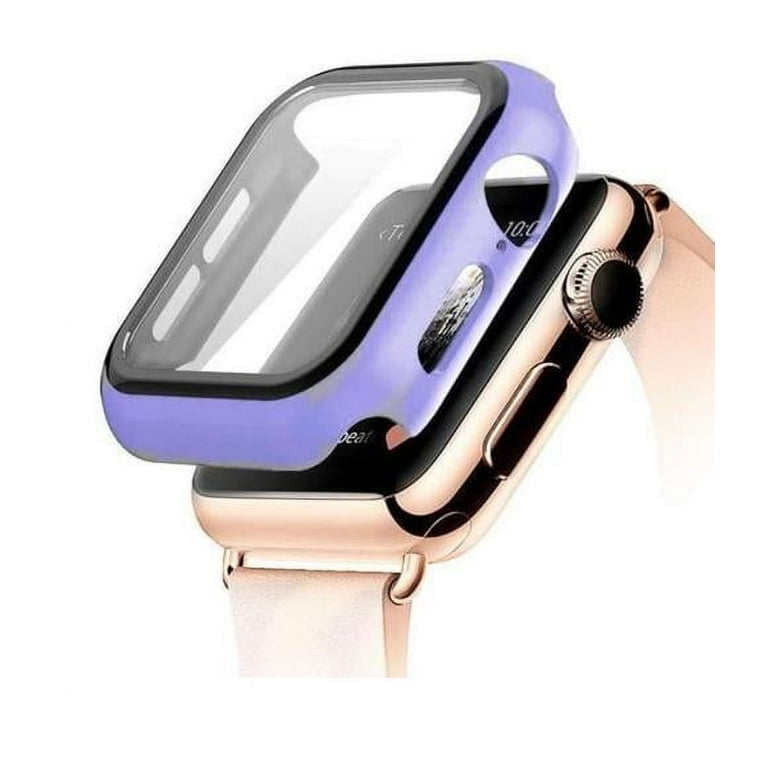The image is a highly detailed, promotional photo of a rose gold Apple Watch with a sleek, rectangular digital face. The watch is adorned with pale pink bands that wrap around buckles on both the top and bottom. The screen displays the time, 10:00, with a "T" in the top left corner and a heart rate indicator at the bottom. Covering the watch is a protective case in a lilac-mauve color with a black border. This case has a transparent front, allowing the screen to remain visible while being shielded from potential damage. The sides feature precise cutouts for the buttons and dials, ensuring a snug fit and ease of access. The cover fits perfectly over the watch, highlighting the care taken in its design. The absence of blemishes or scratches on the smartwatch, combined with the professional composition of the image, suggests that this advertisement is showcasing the cover as an ideal protective accessory for the Apple Watch.